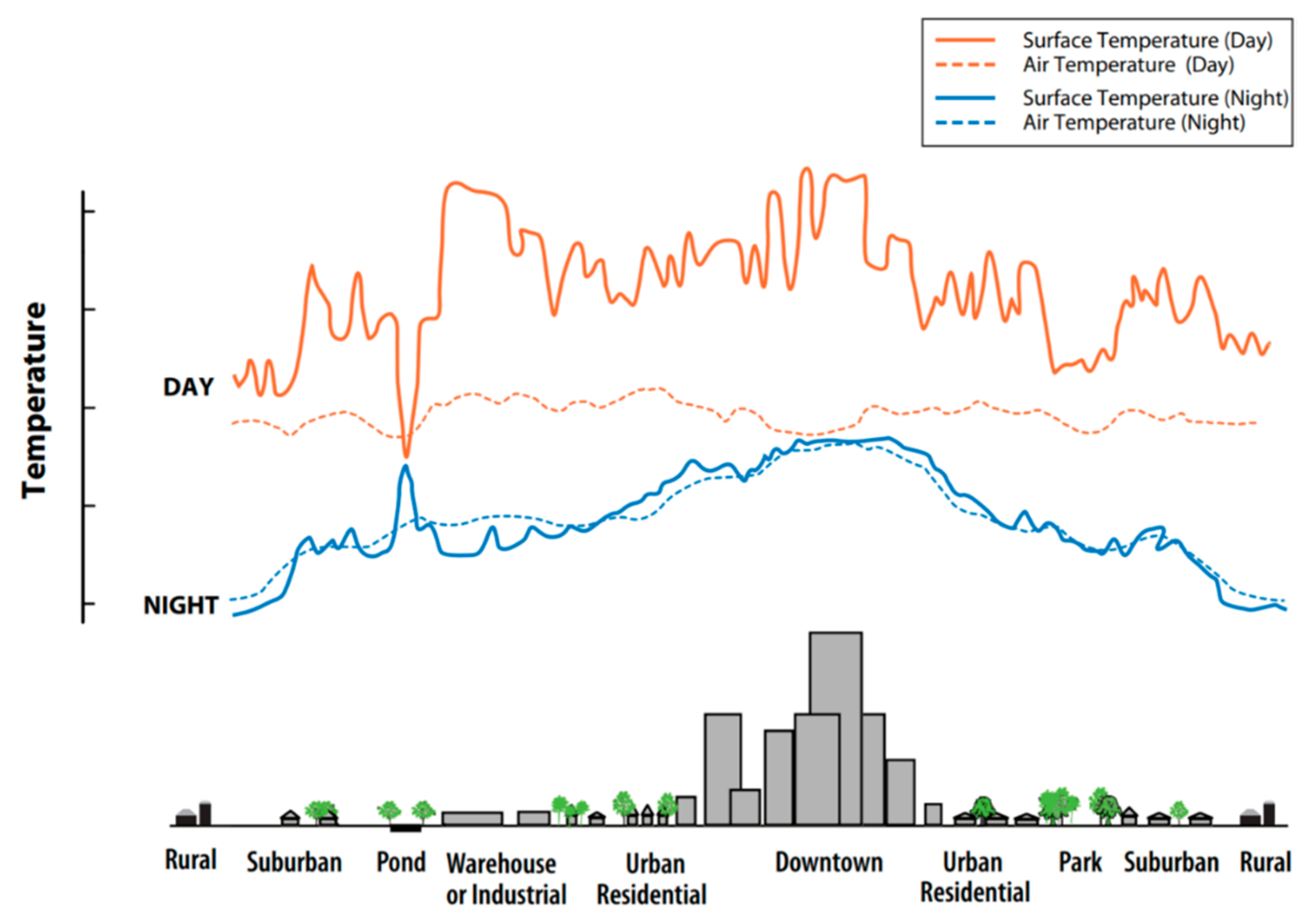The image shows a detailed weather graph comparing surface and air temperatures during the day and night across different areas. The left edge of the chart is labeled "temperature" in black text with a corresponding scale, while the bottom of the chart is labeled with various zones: rural, suburban, pond, warehouse or industrial, urban residential, downtown, urban residential, park, suburban, and rural. The top right corner features a legend with four types of lines: a solid orange line for daytime surface temperature, a dotted orange line for daytime air temperature, a solid blue line for nighttime surface temperature, and a dotted blue line for nighttime air temperature. The graph indicates higher temperatures in downtown and urban residential areas compared to rural areas, both during the day (in orange) and at night (in blue), with the solid lines representing surface temperatures and the dotted lines representing air temperatures.